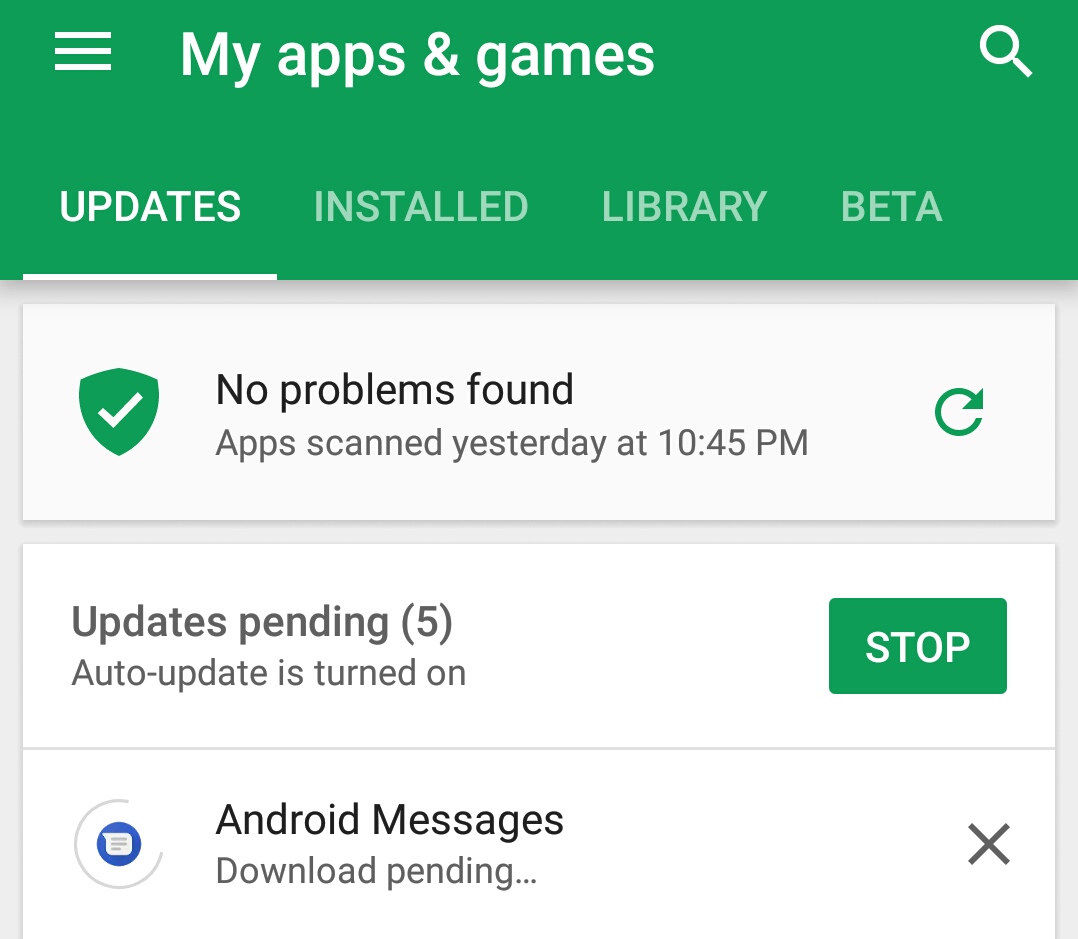The screenshot displays the "My Apps & Games" section within an app interface. The top of the screen is bordered in green and features a hamburger menu icon on the top left, labeled "My Apps & Games." On the top right, there is a magnifying glass icon. Below this, a navigation bar includes tabs labeled "Updates," "Installed," "Library," and "Beta," with the "Updates" tab highlighted and underlined in white.

Beneath the navigation bar, a notification box with a green shield and white check mark states, "No problems found. App scanned yesterday at 10:45 PM." Beside this message, a circular, clockwise arrow suggests a refresh or retry action.

Further down, the text "Updates pending (5)" is displayed, along with a message indicating that auto-update is turned on. Adjacent to this, a green box with white capital letters reads "STOP." 

A division line separates the content above from below. Under this line, a circular icon containing a blue circle and a text box displays "Android Messages download pending..." followed by an ellipsis. An "X" icon is located in the upper right of this section, allowing the user to cancel the download. The remaining part of the screen shows empty space.